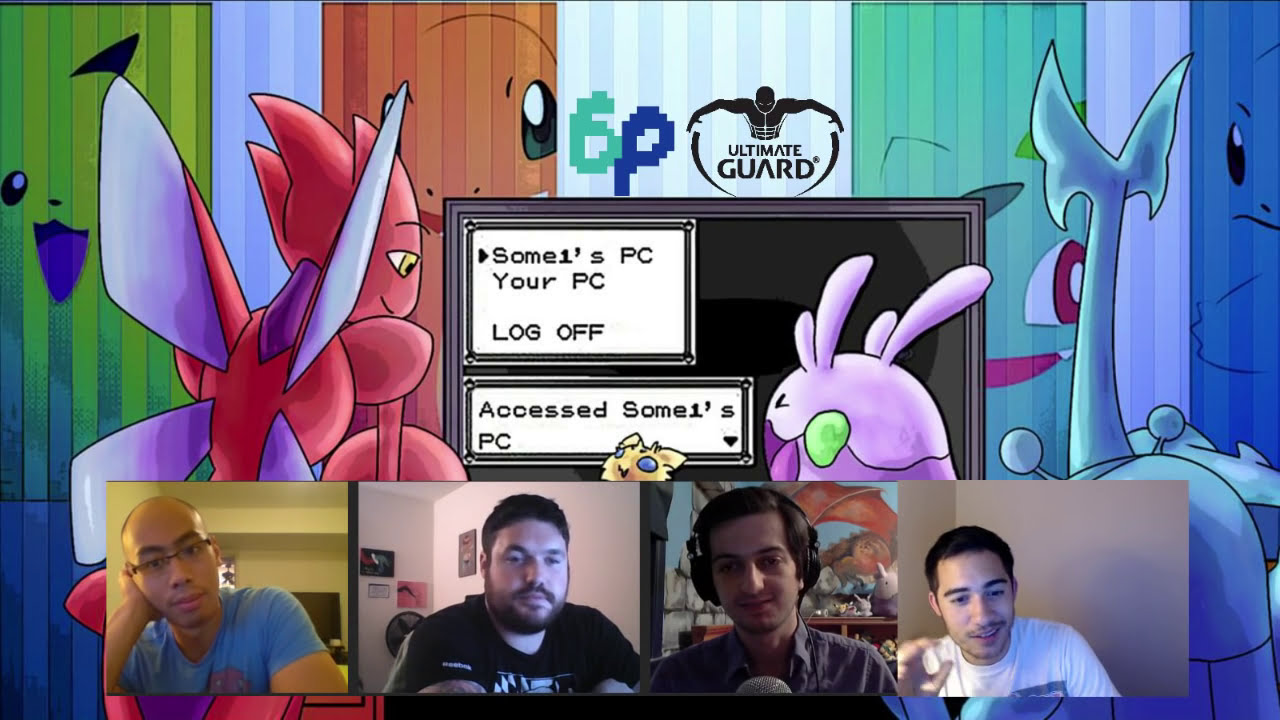The image is a detailed, animated illustration, closely resembling a scene from a child's game or book, with a whimsical, Pokemon-like background. The backdrop features a wall adorned with what appears to be drapes or wallpaper. Prominently displayed are animated, indistinct faces characterized by eyes and tongues but lacking complete facial clarity. This vibrant scene showcases a palette composed of shades of green, white, gray, orange, blue, aqua, reds, white, black, and purple.

In the foreground, there are animated figures, including one described as a red dragonfly-like character accompanied by a few other characters reminiscent of Pokemon, such as Pikachu, Charmander, Bulbasaur, and possibly Venusaur. One notable character has bunny ears, and another has a long neck with axe-like facial features.

Center stage is a gray, TV-like device displaying the text "Ultimate Guard" and "S-o-m-e-o-n-e's PC," followed by "Your PC" and "Logged Off." Below this is a white text box stating "Accessed Someone's PC." 

The lower section of the image features a row of webcam feeds showing four distinct men engaged in what looks like an online live chat or group Skype session, likely discussing or playing a video game. Each participant is in a separate square: a balding Asian man in a blue shirt, a bearded man with short hair in a black shirt, a man wearing headphones and talking into a mic who appears to be of Indian descent, and a young Hispanic man in a white T-shirt. The screen captures a diverse array of users, emphasizing the collaborative and interactive nature of their activity.